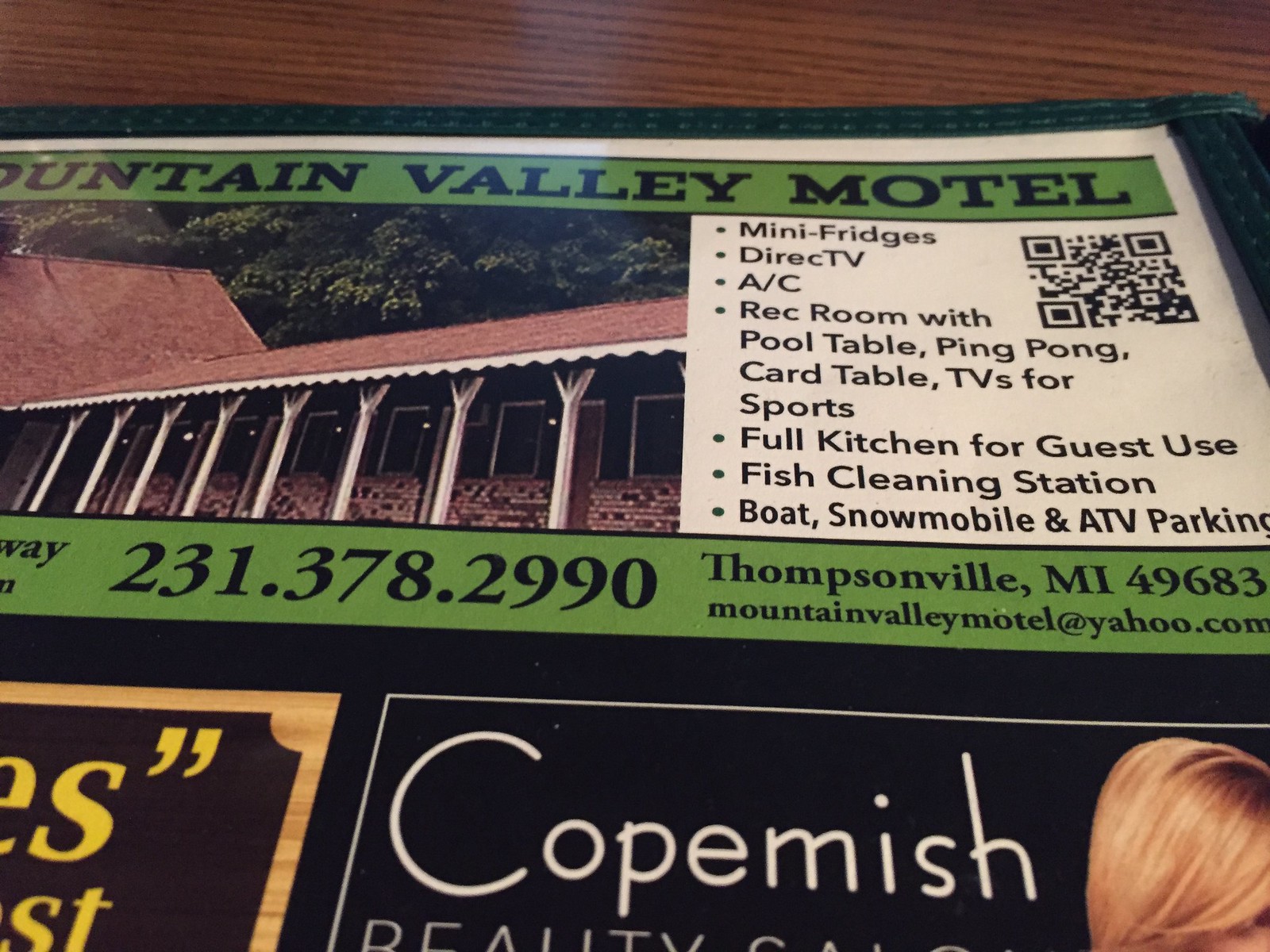The image depicts a detailed color photograph, oriented in landscape, showcasing a large banner sign positioned against a brown wooden surface. The image is a section of a printed publication, featuring a color print advertisement. At the top, the green strip displays the title "Mountain Valley Motel" in black type, accompanied by a photograph of a small, single-floor motel with a distinctive red roof and white columned porch. The contact details are clearly listed: phone number 231-378-2990, Thompsonville, MI 49683, and the email mountainvalleymotel@yahoo.com.

Below the banner, a QR code sits prominently, alongside a comprehensive list of amenities offered by the motel, which includes mini-fridges, Direct TV, air conditioning, a recreation room equipped with a pool table, ping pong, and card table, TVs for sports, a full kitchen for guest use, a fish cleaning station, and parking for boats, snowmobiles, and ATVs. Additionally, part of a separate advertisement for a local beauty salon, "Copemish Beauty," is visible but cut off at the edges.

In the foreground, the back of a woman's blonde head can be seen as she looks up at the signage, adding a human element to the otherwise informational scene. The photograph is a representational realism, highlighting the motel's offerings in a clear and accessible manner.